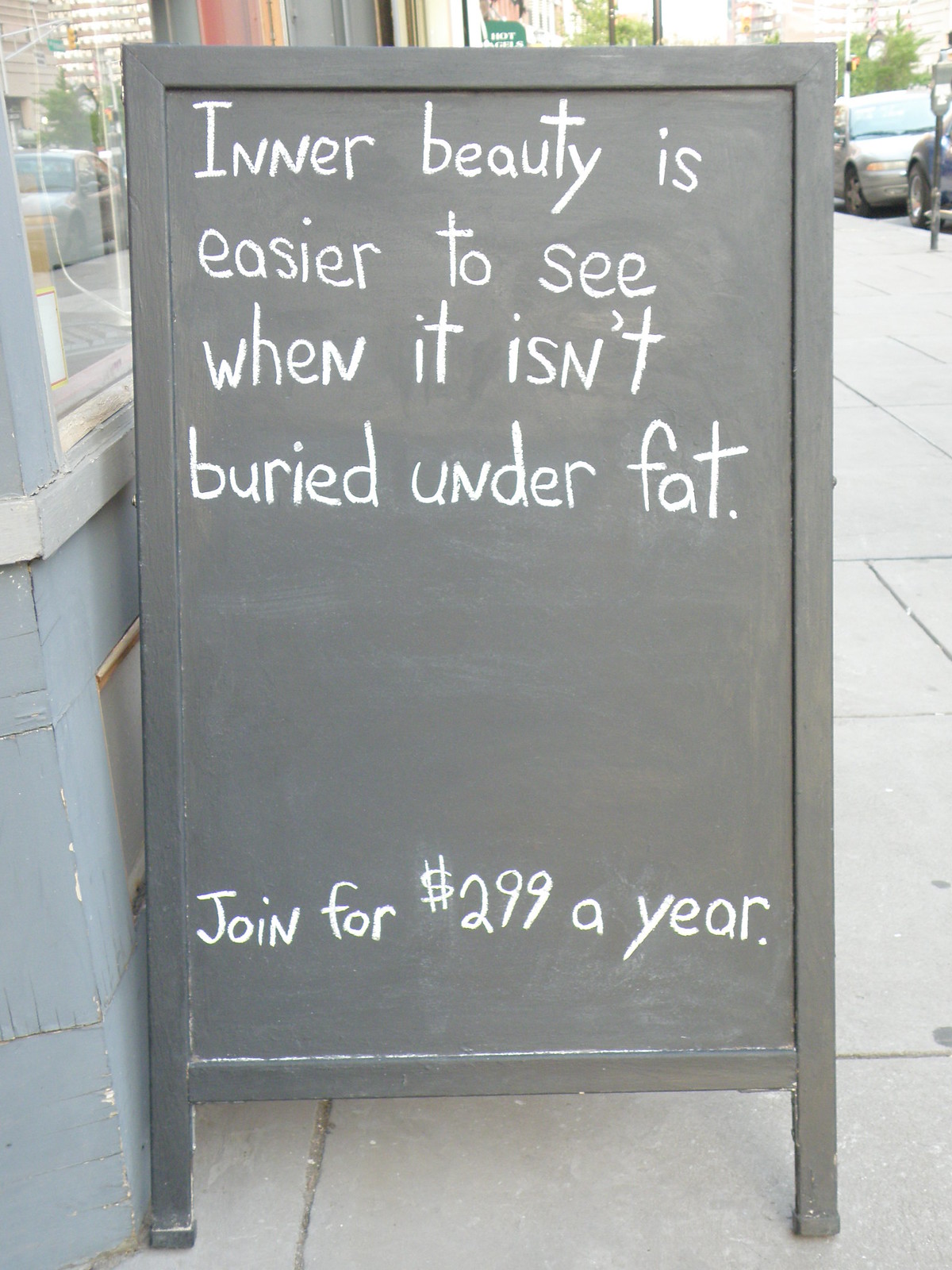The photograph is a rectangular, daytime shot featuring a sandwich board situated on a sidewalk adjacent to a gray, older-looking building on the left. Bright natural light bathes the scene, illuminating parked cars and a visible parking meter on the right. The sandwich board, framed in black with a black chalkboard center, bears a message written in white chalk: "Inner beauty is easier to see when it isn't buried under fat." Below a blank space, the sign continues with: "Join for $299 a year." The handwritten text varies between lowercase and uppercase letters, suggesting an informal, non-professional style. This appears to be an advertisement for a business located inside the building.